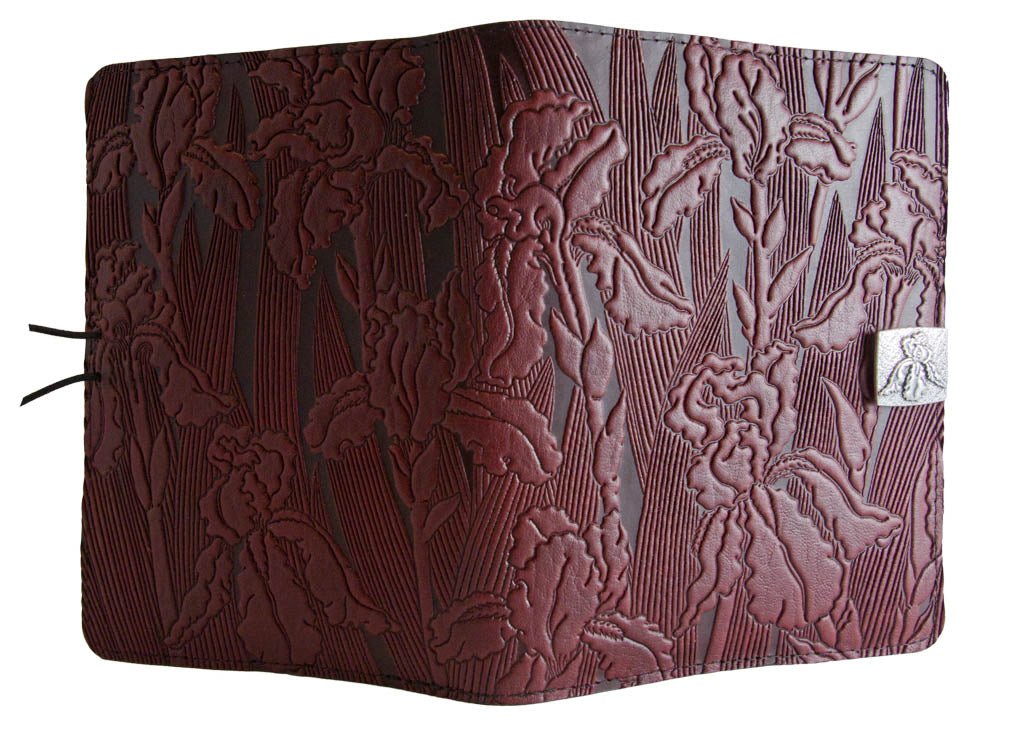The image is a high-resolution color photograph in landscape orientation, showcasing an opened leather-bound notebook or diary. The cover is a rich, dark burgundy leather with an intricately etched floral design featuring stems, leaves, and petals, giving it a textured, raised appearance. The spine of the notebook is positioned towards the viewer, with the back cover on the left and the front cover on the right. A silver buckle clasp adorns the right edge, complemented by a leather tie on the left that secures to the clasp when the notebook is closed. The background has been dropped out, making the notebook appear to float on a pristine white backdrop, enhancing its detailed craftsmanship in a style that is both representational and realistic, fitting for product photography.